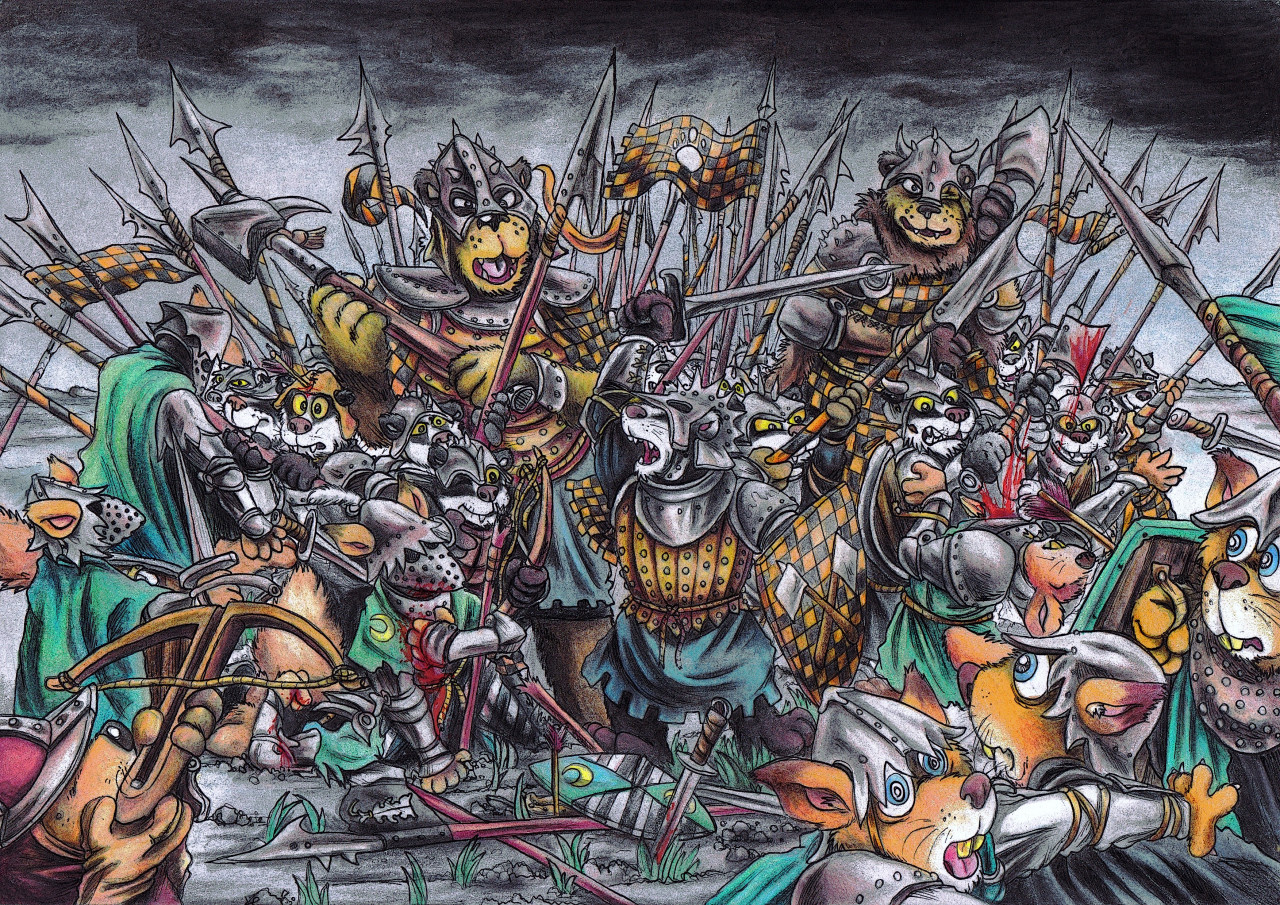In this detailed illustration, predominantly created with markers, we observe a chaotic scene depicting a fierce and bloody battle among anthropomorphized animals, primarily cats, bears, and possibly cheetahs, foxes, or mice. These animated characters are adorned in medieval armor, featuring silver helmets, gold chest plates, and shoulder pads, with some wielding long spears and others equipped with crossbows. The bears stand out due to their considerable height, towering over the other creatures. The scene exudes chaos, reflected in the intense expressions on the animals' faces and the disarray of weapons, including numerous spears scattered across the battlefield. The ground beneath their feet is gray with sporadic patches of grass, while the sky above transitions from a dark gray at the horizon to a near-black hue at the top, encapsulating the somber and intense atmosphere of the battle.